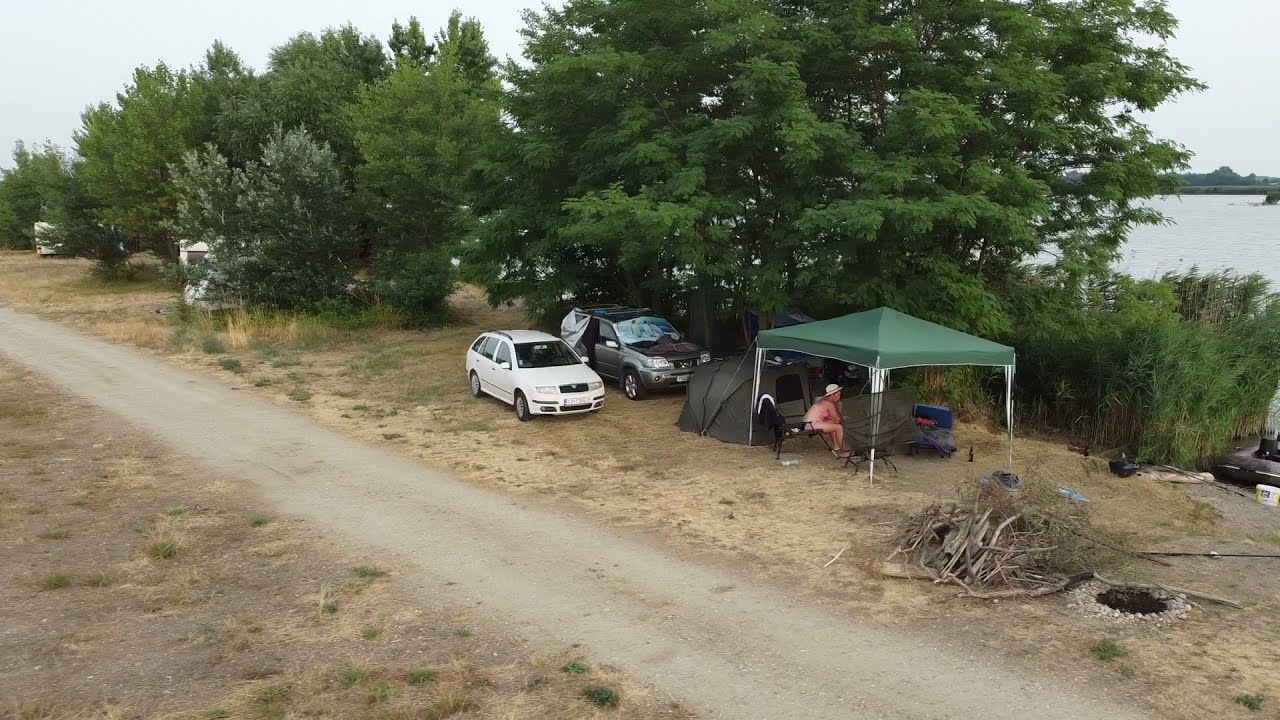In the foreground of the image, a dirt road winds diagonally from the bottom right to the center left. On either side of the road, the ground is littered with dry, brown grasses. Adjacent to the road, under the shade of a large green tree, there is a green-topped canopy supported by four poles, providing shelter for a lady in a pink outfit and a white hat. Nearby, a black dog lounges in the shade. Next to the canopy, a white station wagon and a gray car with an open door and a piece of cloth hanging over it are parked. The gray car also has a reflective sunshade in its windshield.

In front of the canopy lies a pile of dead wood next to a circle of rocks, likely a campfire setup. On the left side of the road, the landscape consists of yellow grass and sparse vegetation. In the background, to the right, there are several trees partially obscuring a light blue body of water, possibly a lake or estuary. The sky above is hazy, adding a muted backdrop to the scene. The overall setting appears to be a rustic campground.